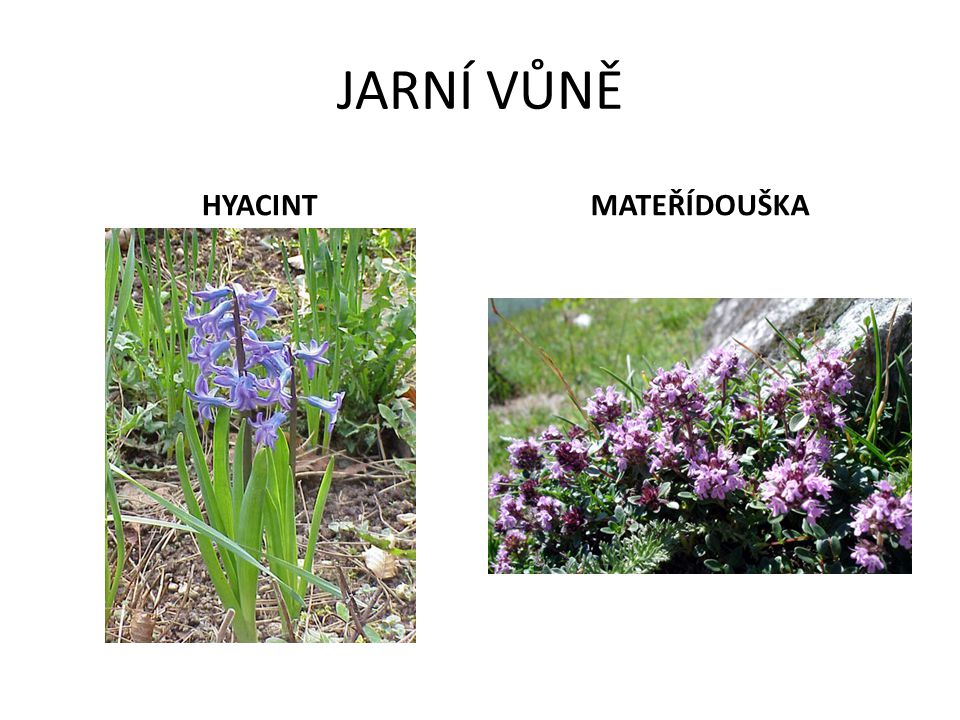These two outdoor photographs showcase flowers in a forest or garden setting during daytime. The first image, arranged in portrait layout, features a hyacinth, labeled "Hyacinth," with around six or seven purple bell-shaped blooms sprouting from green leaves on brown soil. Sunlight illuminates the flowers, highlighting their vivid color against the natural background. In the adjacent landscape mode image, labeled "Materidouska," a cluster of approximately 20 smaller purple-pink blossoms is displayed. These blooms, part of a bush-like plant, are accompanied by thin green leaves, a rock, and some grass in the background. Both images incorporate computerized text on a white background, with the labels and a stylized title, "Jarni Venu," featuring accents over the letters I, U, and E. The hyacinth is depicted with traditional floral elegance typical of spring, while the Materidouska presents a wild, clustered aesthetic amidst the natural surroundings.